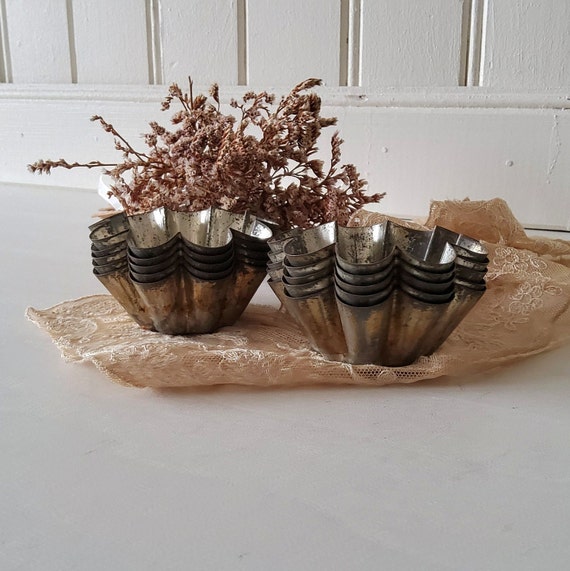This photograph features an indoor setting with a white wall in the background and a gray floor. Central to the image are two groups of bronze and silver hexagon-shaped planters, which resemble metal muffin containers, stacked inside each other, four in each set. Below these planters is a light brown or pink drapery or tablecloth. A potted plant with withered reddish-brown flowers is positioned in the background. The overall scene captures a casual indoor arrangement with a white backdrop, creating a stark contrast against the vibrant, yet slightly faded, elements in the foreground.